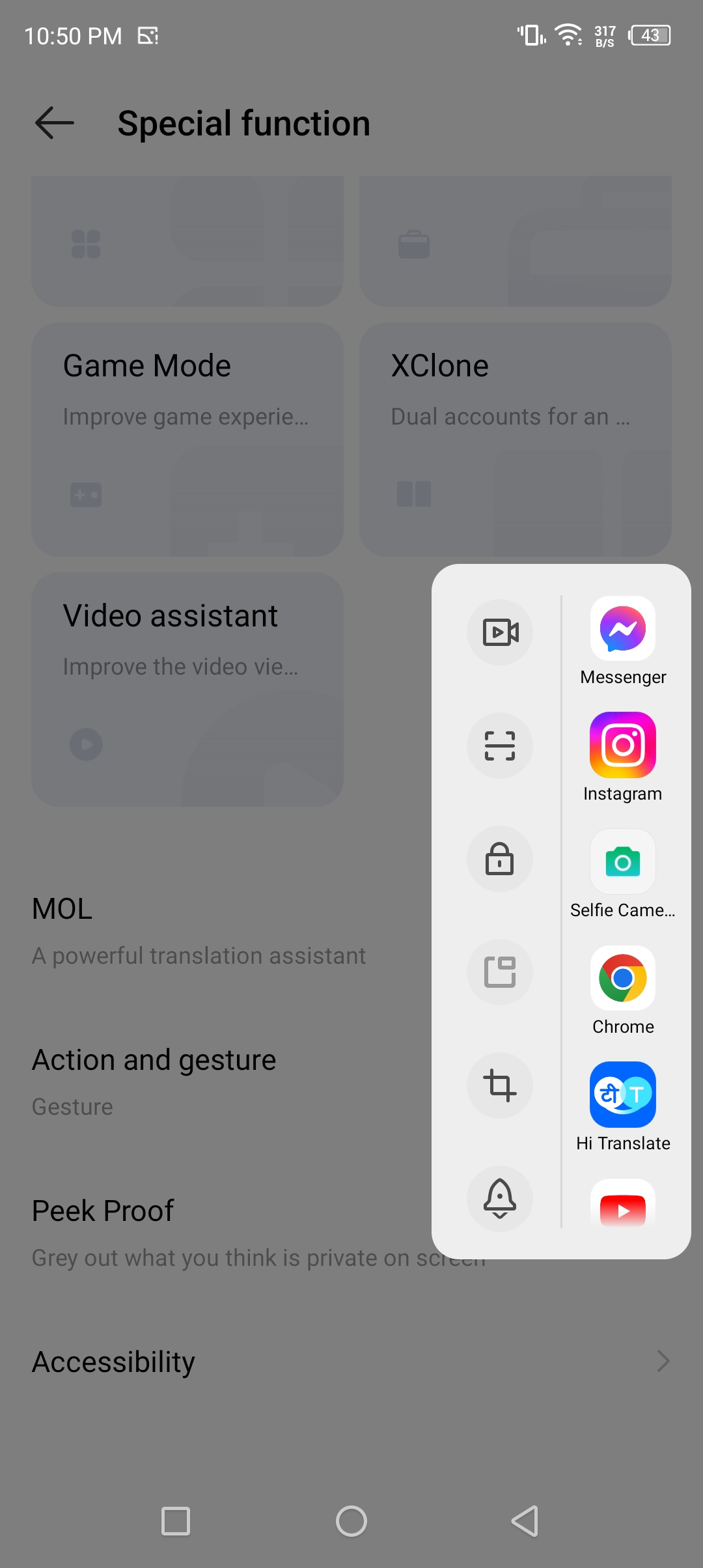In this detailed screenshot taken from a cell phone, the time "10:50 p.m." is displayed in the upper left corner against a gray box in white text. To the right of the time, the status bar indicates the Wi-Fi is on with a speed of "317 B/s" and the battery level at "43%".

Underneath, in black text, we can see "Special Function" with an arrow pointing to the left. Below this, in a light blue box, we find the option "Game Mode" accompanied by the description "Improve game experience". To the right of the "Game Mode" box, there is another similar box. However, the color is gray or light blue and the text reads "X Clone" for dual accounts.

Further below, on the left, there is another light blue box labeled "Video Assistant" designed to "improve the video experience." Finally, at the very bottom are the options for "MOL," a powerful translation assistant, and "Action and Gesture" which includes "Peek Proof" to gray out private content on the screen. This menu interface appears well-organized, presenting various advanced functionalities available on the device.